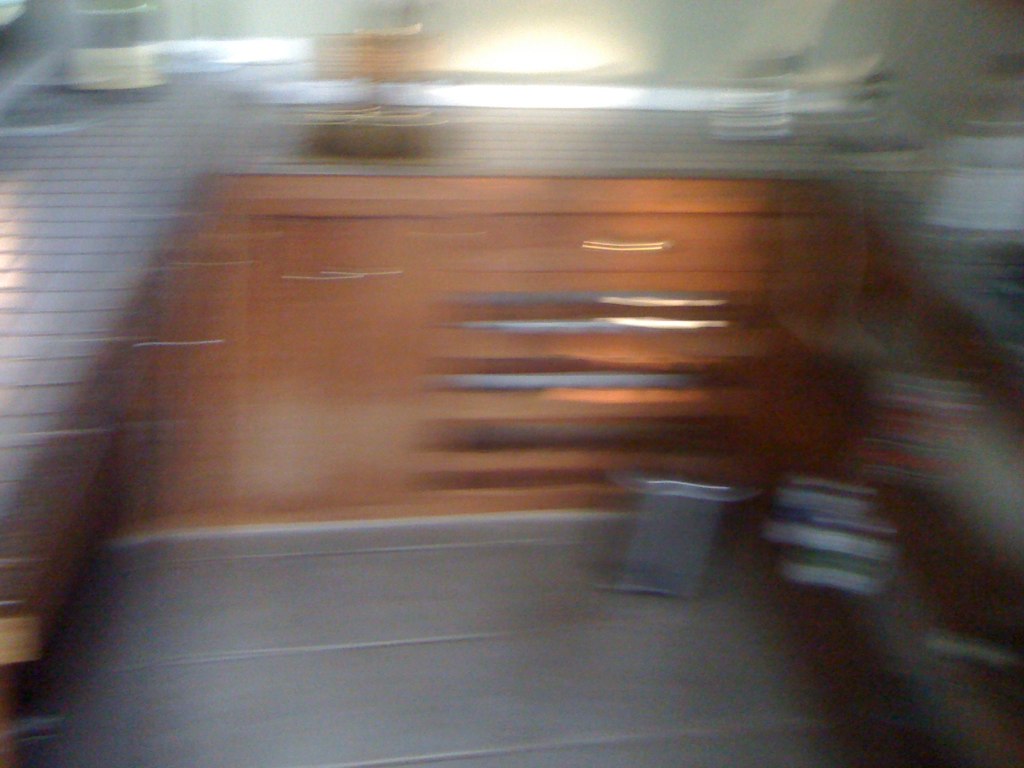This photograph captures the interior of a kitchen featuring a wraparound wooden cabinet with a medium wood finish, highlighting visible wood grains. The cabinetry is outfitted with numerous drawers, each adorned with metal drawer pulls. Though the image is blurry, suggesting motion or a dropped camera, some details are discernible. A gray tiled surface tops the wraparound cabinet, and in the background, there is a sink positioned under a large window with a pull-down, spring-loaded shade. The kitchen floor is laid with medium gray tiles, and to the right, there appears to be a stove or range top.